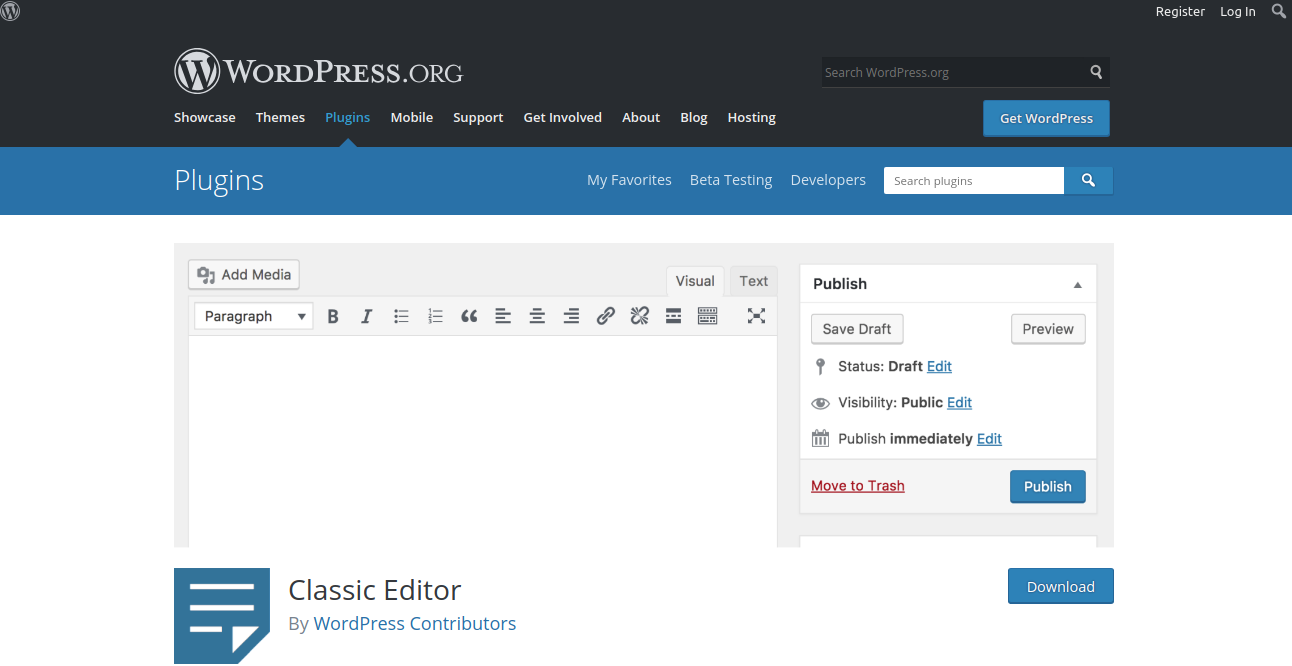The image showcases a webpage from WordPress.org with a detailed view of its interface. At the top, there is a black header featuring the WordPress logo and the text "WordPress.org" in white. Below the header, a navigation menu displays "Showcase," "Themes," "Plugins," "Mobile," "Support," "Get Involved," "About," "Blog," and "Hosting," with "Plugins" highlighted in blue. On the far right side of the header, there's a search bar and a blue "Get WordPress" button. Additionally, the top right corner includes options for "Register," "Log In," and a search icon.

In the main content area, below the highlighted "Plugins" section, there are more navigation options, including "Plugins," "My Favorites," "Beta Testing," and "Developers." To the right, there is a search bar with a search icon labeled "Search Plugins."

Further down, there's a user interface section with a white button labeled "Add Media." It includes a headline input field or a header dropdown menu for formatting text. This section includes various stylistic buttons for different text styles. On the far right, there's a box labeled "Publish," featuring options such as "Save Draft," "Preview," and status updates of the content. Below these options, there is a blue "Publish" button, a blue "Download" button, and an adjacent page icon labeled "Classic Editor by WordPress Contributors."